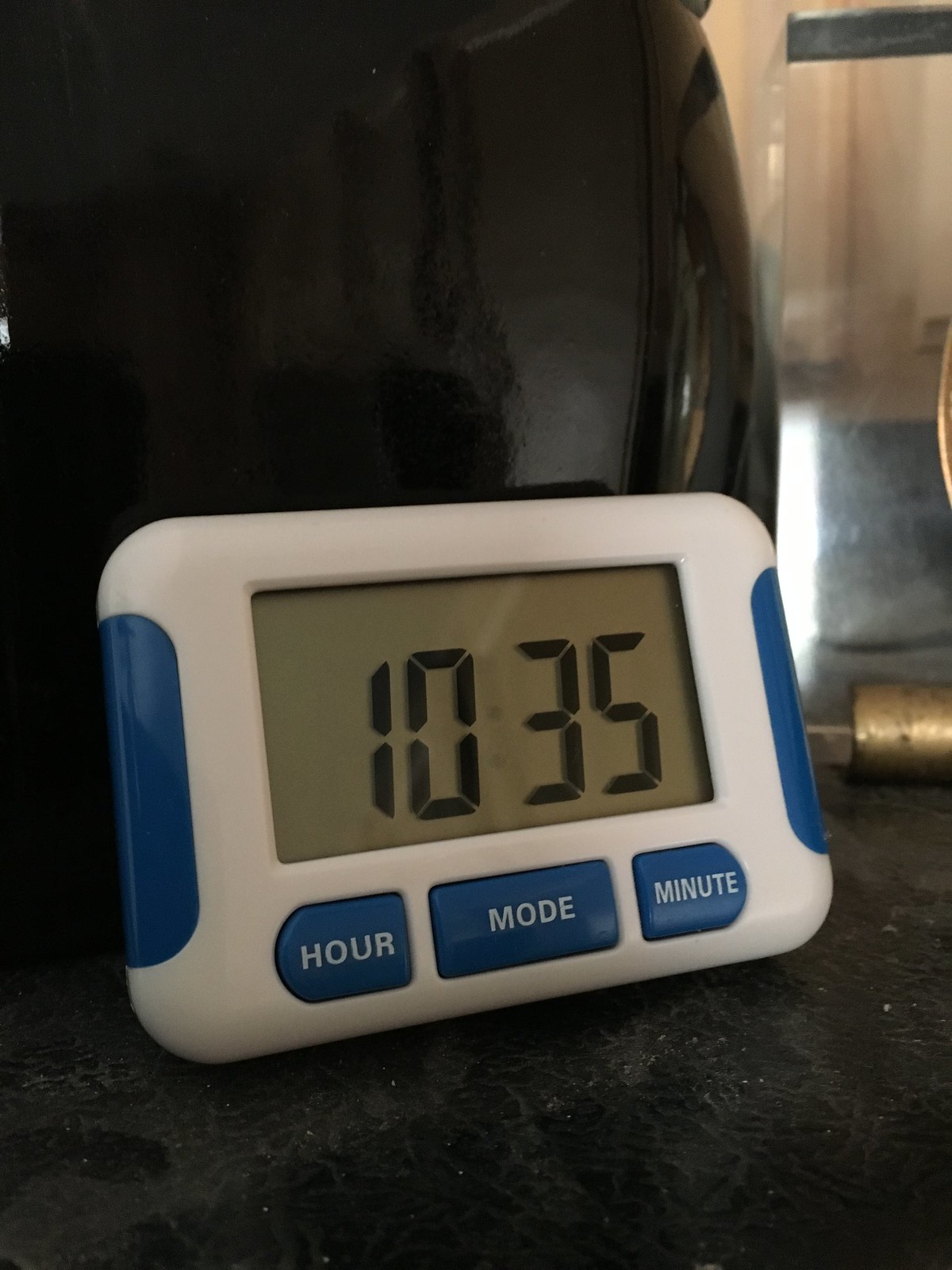This detailed image captures a white-framed digital clock with a sturdy back resting on a blurred surface, likely a desk or kitchen table. The clock’s sides are medium blue, with matching blue buttons at the bottom. The outer buttons are oval-shaped with flat tops and bottoms, labeled "hour" and "minute" in white, while the middle button is rectangular, labeled "mode". The digital screen has a brownish-tan background displaying the current time, 10:35, in black digits. The clock is positioned against a brown cabinet background, with a blurry black object partially visible behind it, ensuring the viewer's focus remains on the clock.